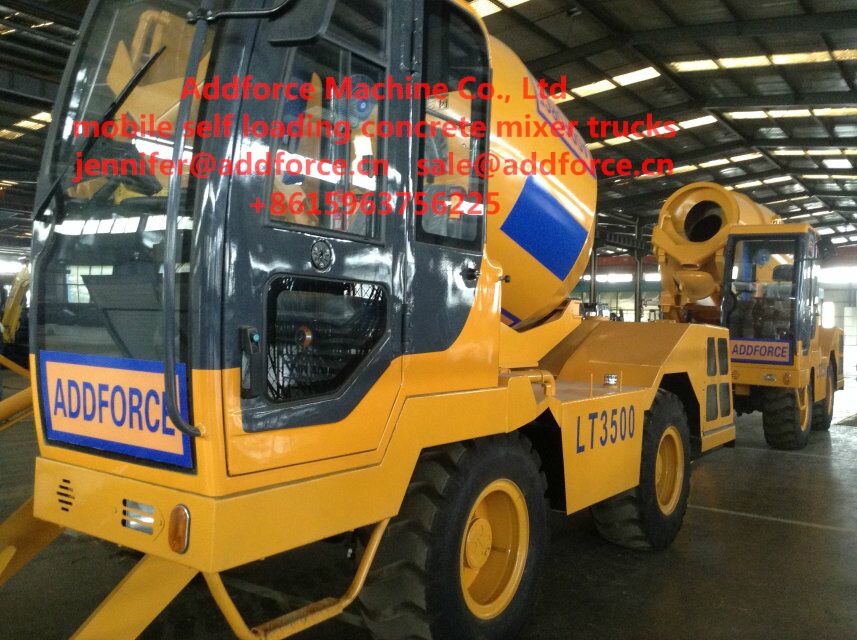The image, in landscape format and color, captures two large, very yellow construction machines identified as self-loading concrete mixer trucks from ADFORCE MACHINE CO. LTD. The vehicles, parked inside a spacious metal warehouse with a concrete floor and fluorescent lighting, boast robust build quality with completely encased, single cab driver compartments made of steel and glass. Each truck is labeled with "LT3500" between the wheels and features notable design elements like a small bucket, large tires, a windshield wiper, and an orange reflector. The front of the trucks displays the ADFORCE logo in blue, with additional labeling in red text overlaying the top of the photo, stating, "ADFROCE MACHINE CO. LTD. Mobile Self-Loading Concrete Mixer Trucks." Contact details for inquiries are provided: Jennifer at ADFORCE.CN, sales at ADFORCE.CN, and the phone number +861-596-375-6225.